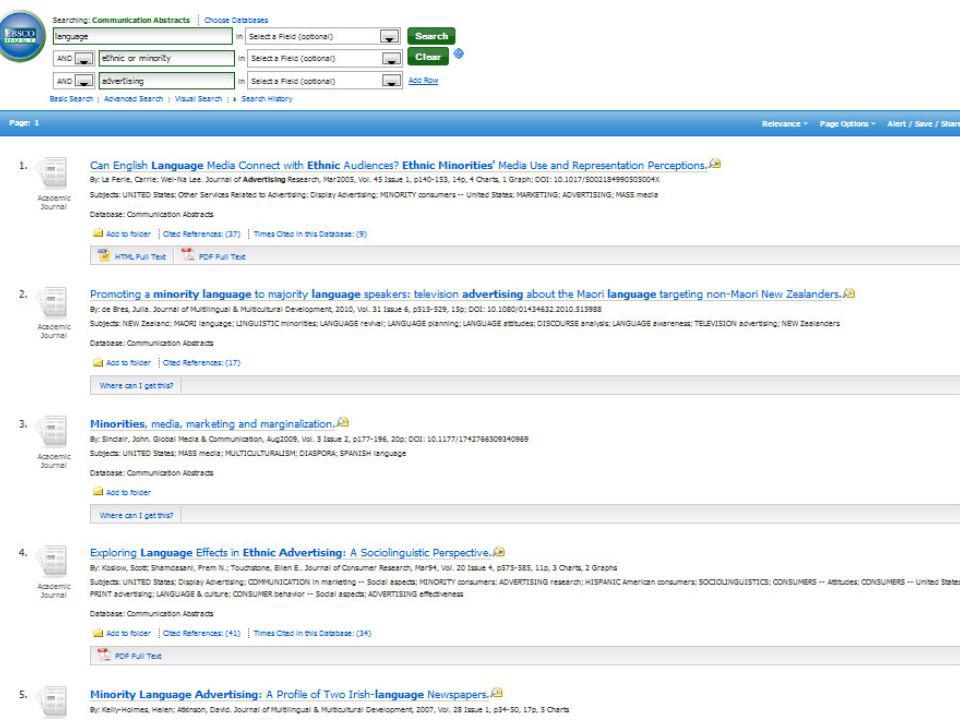The image depicts a digital form with a somewhat cluttered layout. At the top of the page, there is a search bar where the word "language" has been entered. Users have the option to select a specific field, though it seems this option was left unselected in this instance. Below the search bar, there are three fields that have logical operators: "Language AND Ethnic OR Minority AND Advertising." 

The main section of the page is more readable and prominently features a list of five academic journals related to ethnicity, language, and marketing. The titles of these journals include topics such as "Can English Language Media Connect with Ethnic Audiences?", "Promoting a Minority Language," and "Minorities, Media, and Marketing," among others. An icon resembling a newspaper, labeled "Academic Journal," appears on the left side of this list. The overall theme of the content focuses on the intersection of language, minority groups, and marketing strategies.